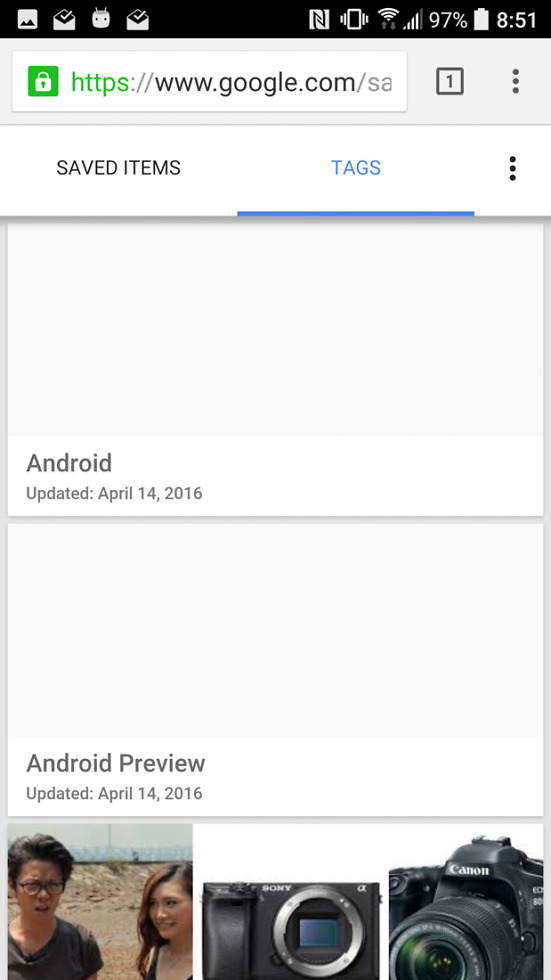The image displays a smartphone screenshot with a black border at the top. In the top-left corner, there are four unidentified icons. On the right side of the black border, the status indicators are visible: a Wi-Fi icon with 4 out of 5 bars, a battery icon showing 97% charged, and the time displayed as 8:57. Below this, there's an address bar featuring a green square with a lock icon in the center, indicating a secure connection. The URL, shown in the address bar, begins with "HTTPS" in green followed by "://www.google.com/SA" in black text.

Beneath the address bar, the text "Save Items" is displayed, followed by "TAGS" in blue uppercase letters with a blue underline. Below this, there's an empty gray area, and a small white rectangular box with the text "Android updated April 14, 2016". Further down, another empty gray area is followed by a second white box stating "Android preview updated April 14, 2016". At the bottom of the image, there are three smaller pictures. The first picture on the left depicts two people, while the other two pictures to the right show a camera.